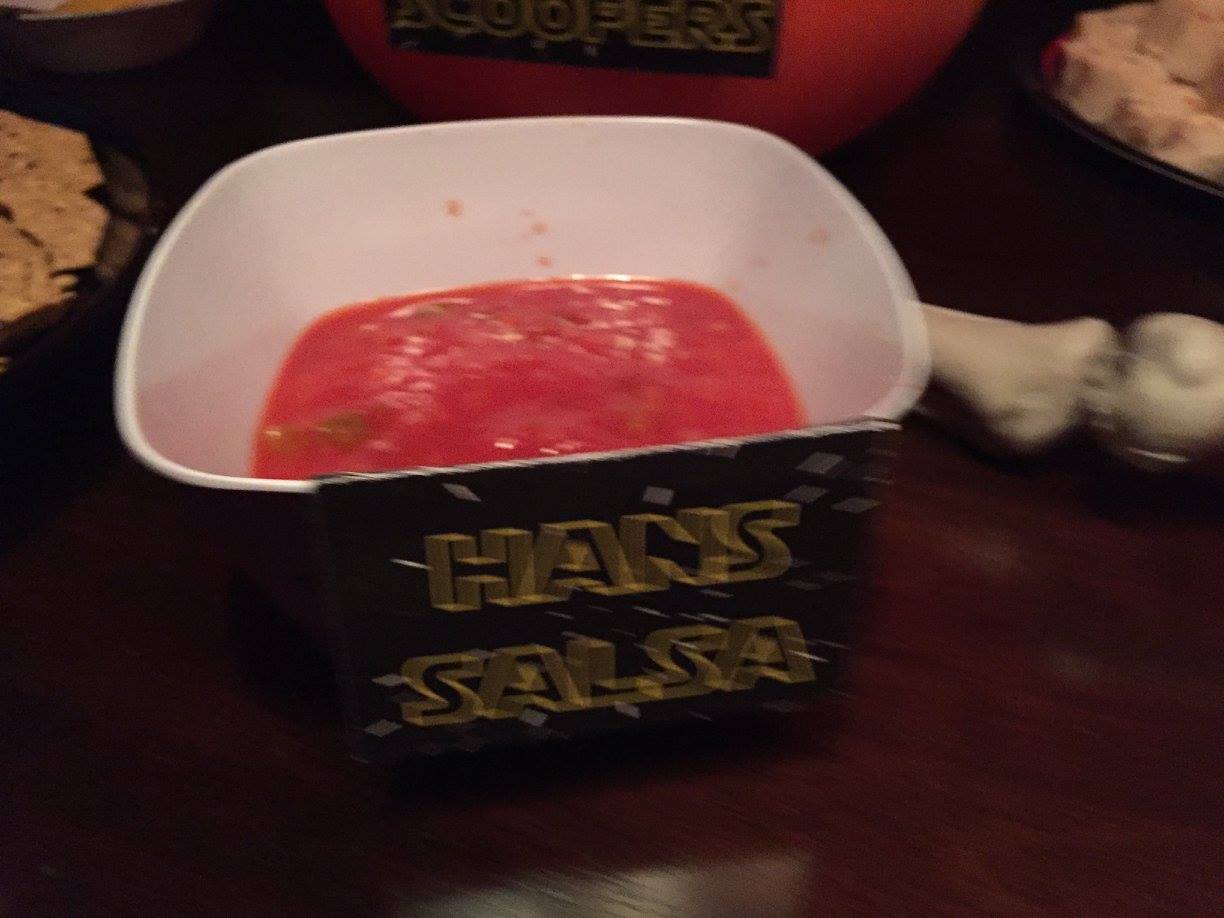The image shows a white, square bowl with a label on the front. The black label features a diamond design and contains black writing that says "Hans Salsa" and "Gold Shadows." Inside the bowl is a red sauce filling about a third of the bowl. Behind the bowl, there are plates of various kinds of food, one of which is a black plate with a white object on it. Additionally, there is another red bowl with a black label stating "Scoopers," outlined in gold. The scene appears to be set on a reddish cherry wood table, adding a warm background to the slightly blurry photograph.